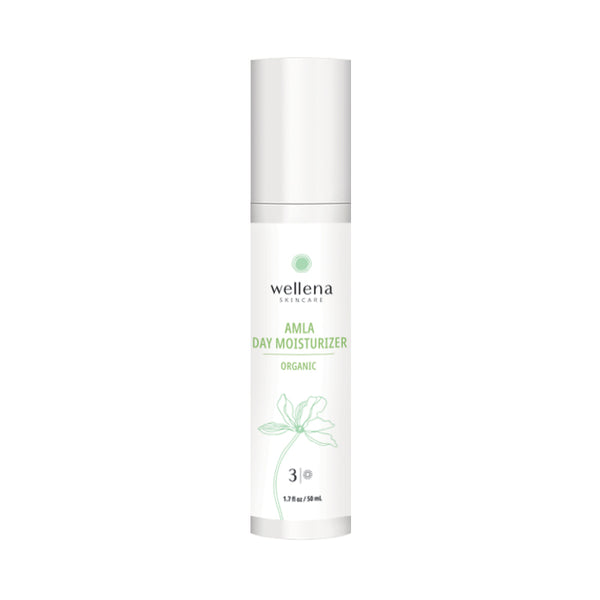The image showcases a cylindrical, silver-gray cap bottle of Wellena Skincare's "Amla Day Moisture" day moisturizer. The bottle features a white label centered on its surface. At the top of the label, a green logo resembling a spiral catches the eye, followed by the brand name "Wellena Skincare" in a bold black font. Below this, in a smaller, teal font, are the words "Amla Day Moisture," underlined by the bold, uppercase word "ORGANIC." A delicate, green outline of a flower with petals extends beneath the text, followed by a black number "3" and a small logo resembling the sun. At the bottom, the product's volume is clearly stated as 1.3 fluid ounces (54 milliliters). The product is set against a plain white background, giving it a clean and modern advertising feel.